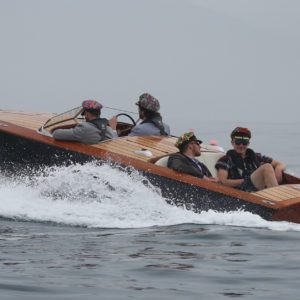In this small, closely-cropped photograph, four middle-aged men are aboard a sleek, vintage-style motorboat—likely a cigarette boat—gliding swiftly over a calm, dark expanse of water. The polished and waxed teakwood (or redwood) planks gleam despite the overcast, grayish sky overhead. The boat, tipped slightly upward at the front due to its high speed, lacks visible landmarks, suggesting an open lake or ocean setting.

Two men, both sporting colorful captain's hats and sunglasses, are positioned in the driver's section, with the driver on the right and a passenger on the left. The rear bench seats accommodate two more men, who are deep in conversation, facing away from the driver and passenger. The entire scene captures a moment of leisurely adventure, the boat's wake creating a dynamic contrast against the placid body of water.